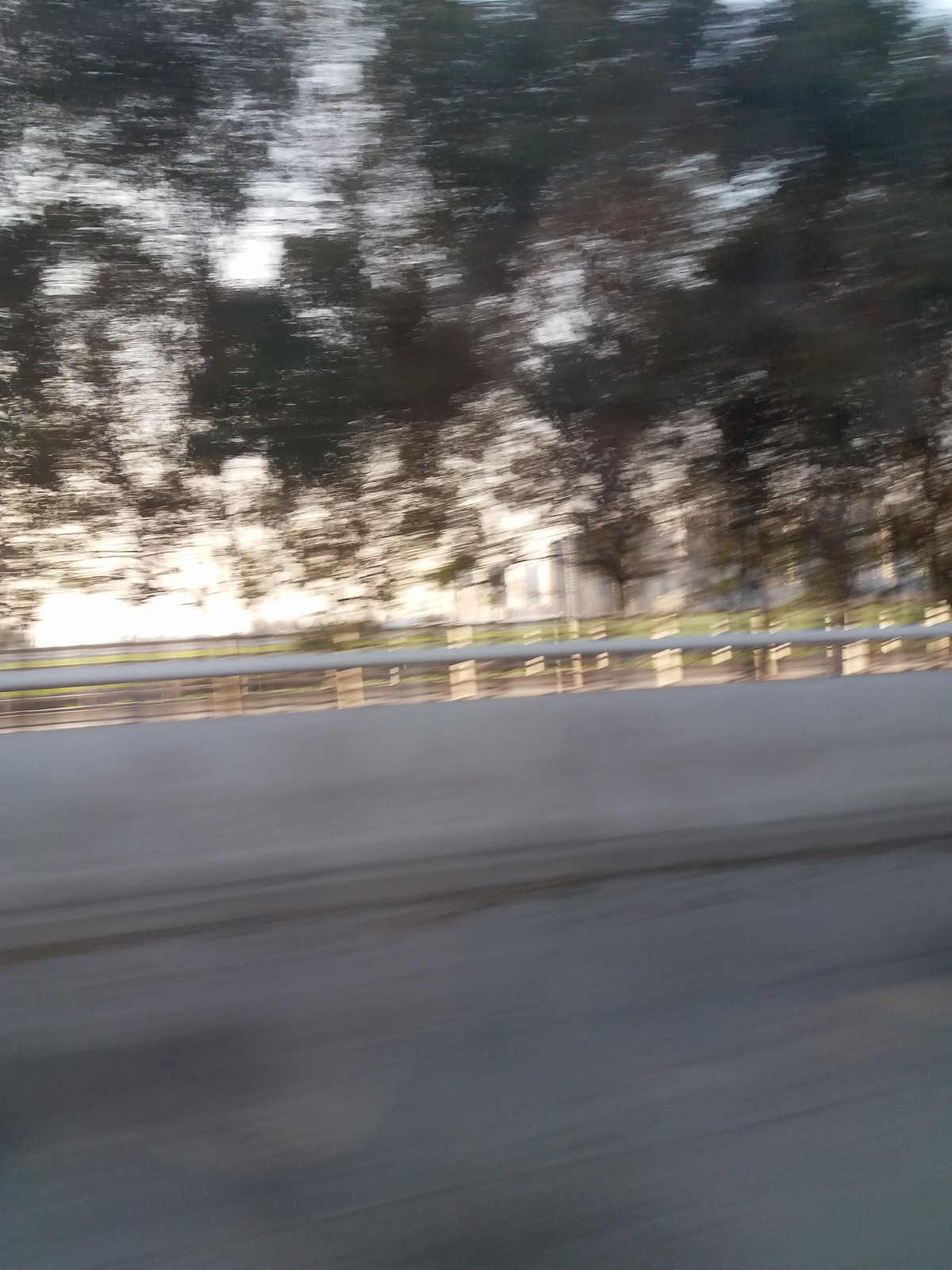This image captures a blurry stretch of a highway, illustrating a segment of the road rather than an extensive view. The highway itself is a medium to dark gray, accompanied by a notably tall median of similar gray shade, with a pole crossing over its top. In the background, there appears to be a building structure, possibly a parking garage or storage units, with its horizontal lines intersected by an overlay of dark green tree leaves, which dominate the upper portion of the image. The photograph suggests motion, as if taken from a moving vehicle, contributing to the overall blur. There's a noticeable contrast where light beams pierce through the leaf canopy, adding pockets of illumination to the scene.